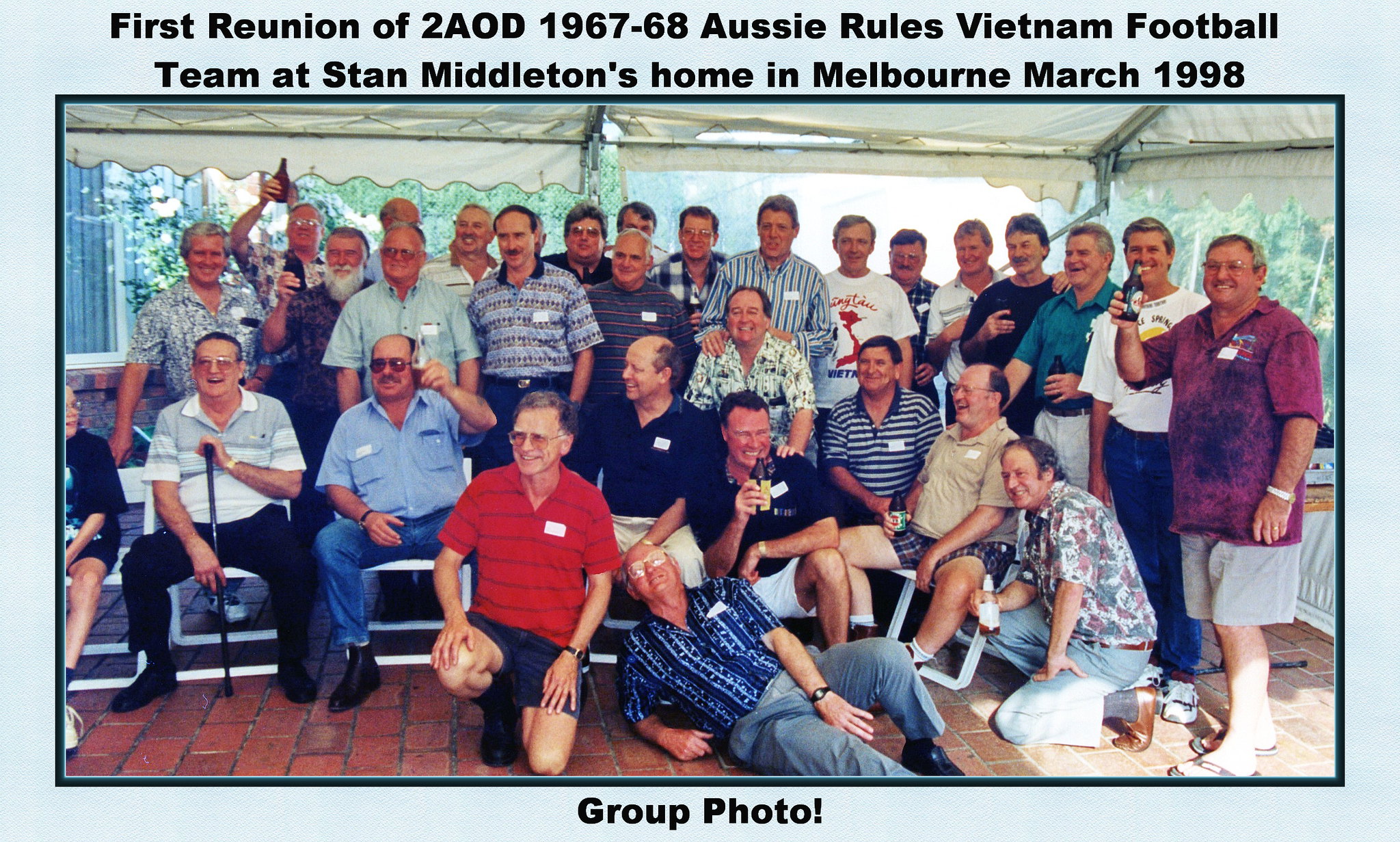This group photo captures the first reunion of the 2AOD 1967-1968 Aussie Rules Vietnam football team held at Stan Middleton's home in Melbourne, March 1998, as indicated by the caption at the top. The setting shows a light blue border framing the image and a red paver or brick platform on which the group is gathered. The men, primarily in their 50s and 60s, are posing casually; some are standing while others are sitting or even lounging on their sides, propped up on their elbows. Many individuals are seen holding drinks, adding to the relaxed atmosphere. They are dressed in a variety of casual clothing, including red and black striped shirts, collared polo shirts, t-shirts, shorts, and casual pants, and most are wearing name tags. In the background, an awning is visible, providing shade for the group. At the bottom of the photo, the words "group photo" are inscribed.